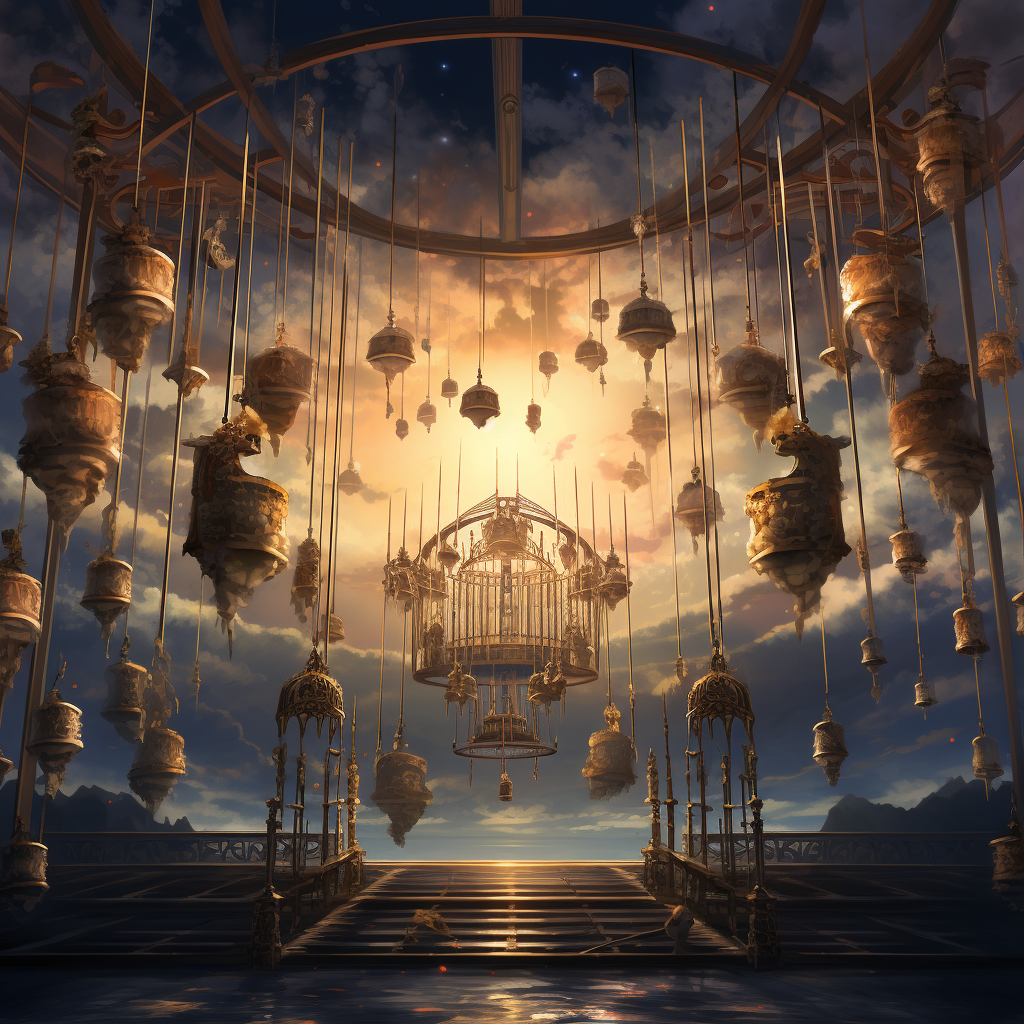This illustration, likely created through digital art or AI, presents a captivating fantasy scene set in the sky. Dominating the center is a prominent, golden birdcage with a conical top and a more bell-shaped lower section. This primary cage, uncluttered within, is surrounded by dozens of similarly structured, cylindrical bell-like cages, all possessing a metallic brass, gold, or bronze finish. These additional cages are suspended by metal poles or strings from a larger, intricate metallic circular structure overhead, resembling a scaffolding system. 

The scene exudes a blend of futuristic and ancient aesthetics, enhanced by a bright light source in the background and partially obscured mountain range. The foreground, possibly depicting a sky boat or plane, is linked to this ethereal sky world. The overall setting, devoid of any visible living creatures, evokes an RPG fantasy environment, hinting at a place where epic boss battles might unfold. The detailed craftsmanship of the cages and the surreal nature of the scene transport the viewer into an unfamiliar, otherworldly domain.